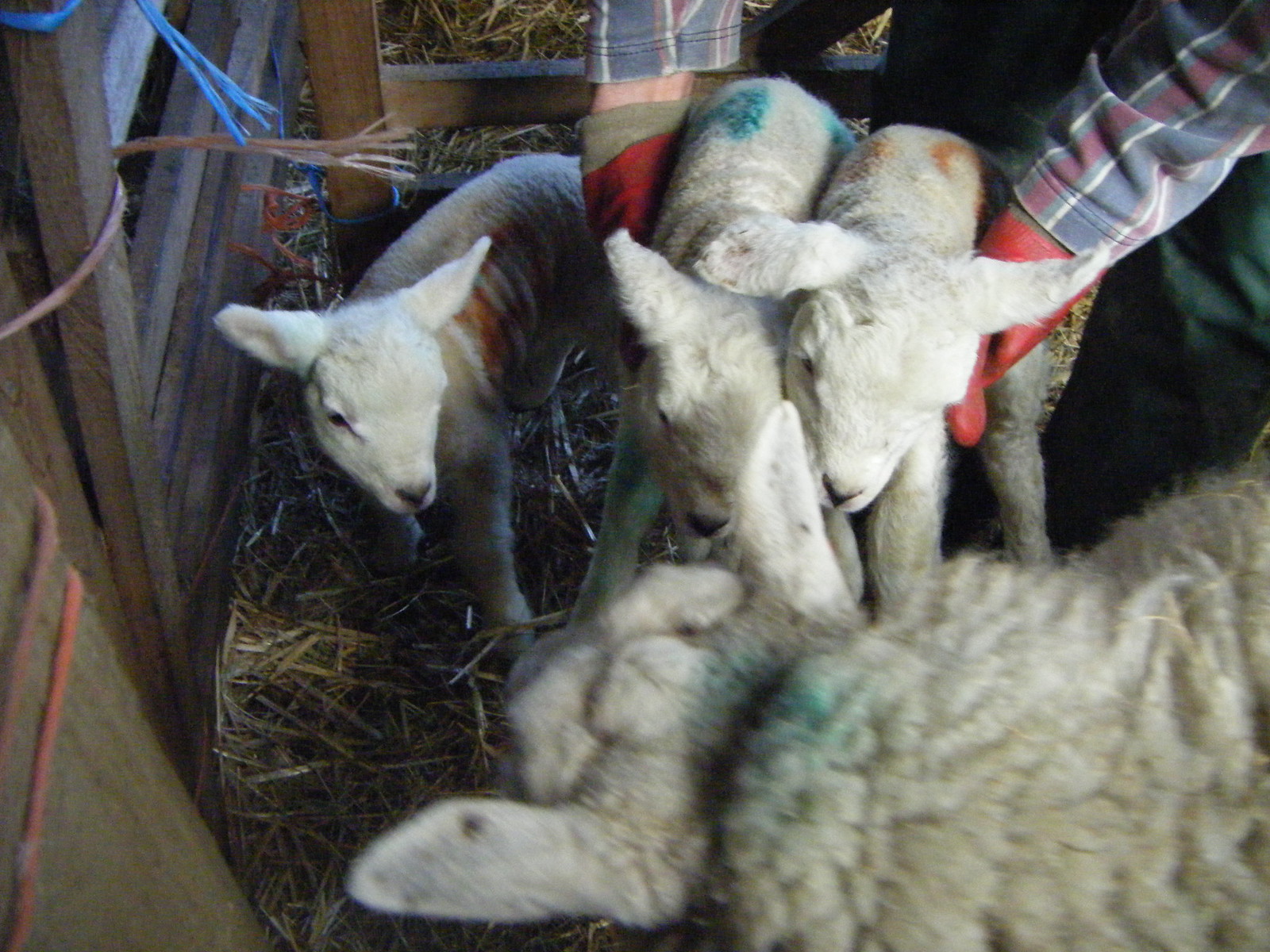In this vivid farm photo, three baby goats, each marked with distinct color stains—two with orange spray and one with blue—stand in the foreground on a thick bed of hay inside a barn. Their pristine white fur contrasts with the vibrant stains, while a full-size goat, possibly the mother, sporting a blue stain on its head, stands at the bottom right corner, turned towards the young ones. Beside the goats, a farmer, whose upper half is obscured but identifiable by the red gloves and a blue-and-red striped shirt, appears to be gently handling the kids. The barn's rustic setting is accentuated by wooden fences secured with varied strings—blue, brown twine, and red elastic—creating a makeshift pen.